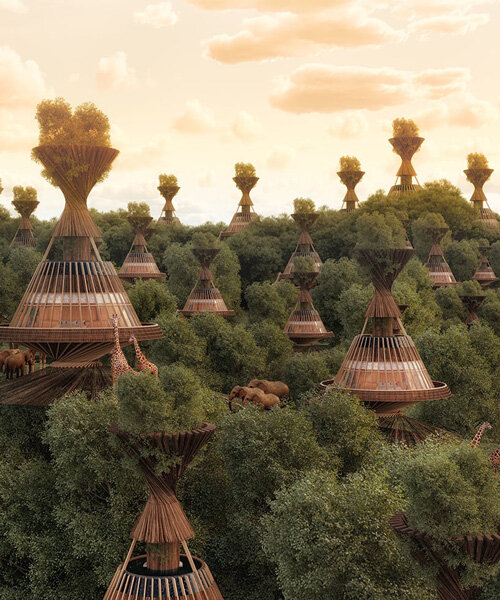The image depicts a tranquil African resort nestled within a lush forest, presenting an elevated camping experience in treetop tent structures. These cylindrical, teepee-shaped tents, crafted from wood, dot the forest landscape repetitively—appearing 11 to 15 times—blending seamlessly with the verdant surroundings. Majestic giraffes and elephants roam freely among the tents on the forest floor, adding a touch of the wild to this unique lodging experience. The scene is bathed in the warm, golden light of a sunrise or sunset, casting an amber hue across the white, cloud-streaked sky. The predominant colors include greens from the abundant foliage, the earthy browns of the tents and forest floor, and a pale white and yellow from the sky. The overall atmosphere evokes a serene, nature-immersed getaway in the heart of Africa.